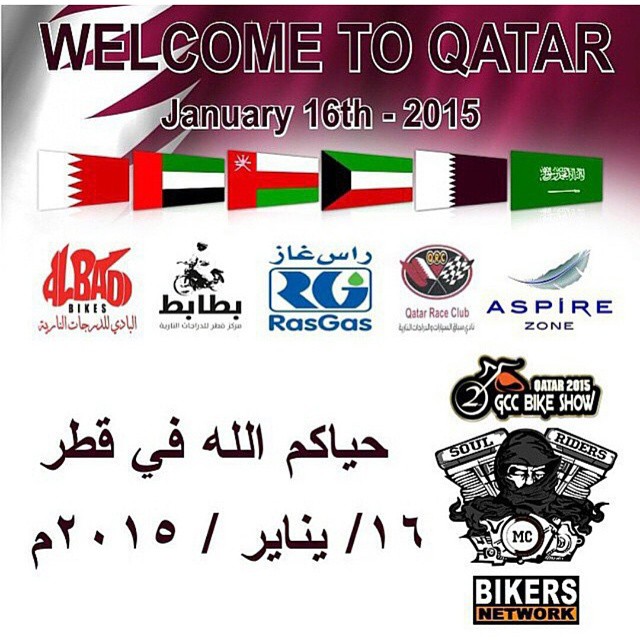The image is a promotional graphic for the Qatar 2015 GCC Bike Show event, held on January 16th, 2015. The upper section prominently features a slogan "Welcome to Qatar" in bold black text with a thin white border, followed by the event date in slightly smaller text. The background of this upper part incorporates the Qatari flag, showcasing a maroon zigzag pattern adjacent to a white field, which gives a dynamic, spiked visual effect on the right.

Beneath the welcoming message is a row of six flags representing Middle Eastern countries. The first flag is half white and half red, likely symbolizing Bahrain, followed by another flag combining red, green, white, and black colors which resembles the Palestinian flag. The remaining flags appear to be from various Middle Eastern nations, including Saudi Arabia.

The lower half of the image, set against a white background, is adorned with numerous logos of sponsoring organizations and clubs. Notable logos include the Qatar Race Club, Al-Bad Bikes, Aspire Zone, and the Soul Riders MC. The Soul Riders logo features an engine graphic with a man wearing a headscarf. Another prominent logo reads "Qatar 2015 GCC Bike Show." Additionally, there is some Arabic text and other smaller logos scattered, enhancing the graphically rich and culturally infused composition of the banner.